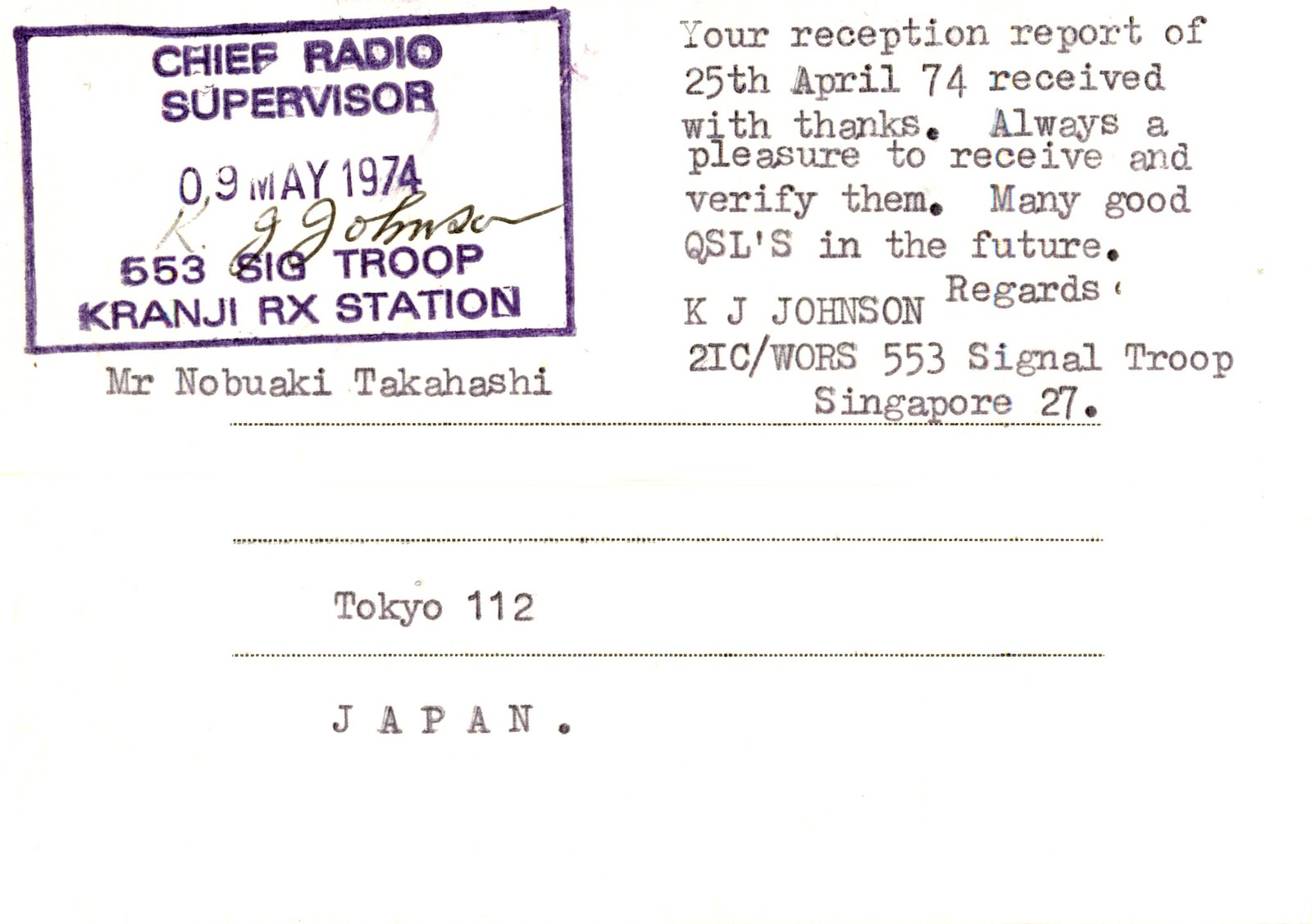The image depicts a document set against a white background. In the upper left corner, there is a blue stamp that reads, "Chief Radio Supervisor, 09 May 1974," with a signature from "G.G. Johnson" underneath. The stamp further states, "553 Sig Troop, K-R-A-N-J-I-R-X Station." Below the stamp, the document features a typewritten message in black font that states: "Your reception report of 25th April '74 received with thanks. Always a pleasure to receive and verify them. Many good QSL's in the future. Regards, K.J. Johnson, 2IC/WORS, 553 Signal Troop, Singapore 27." Beneath the message, the name "Mr. Nobuaki Takahashi" is typed, followed by "Tokyo 112," and "Japan" written in all capital letters. The overall layout has address lines, and an organized, typewritten format, which might indicate the document is related to a telecommunications exchange.